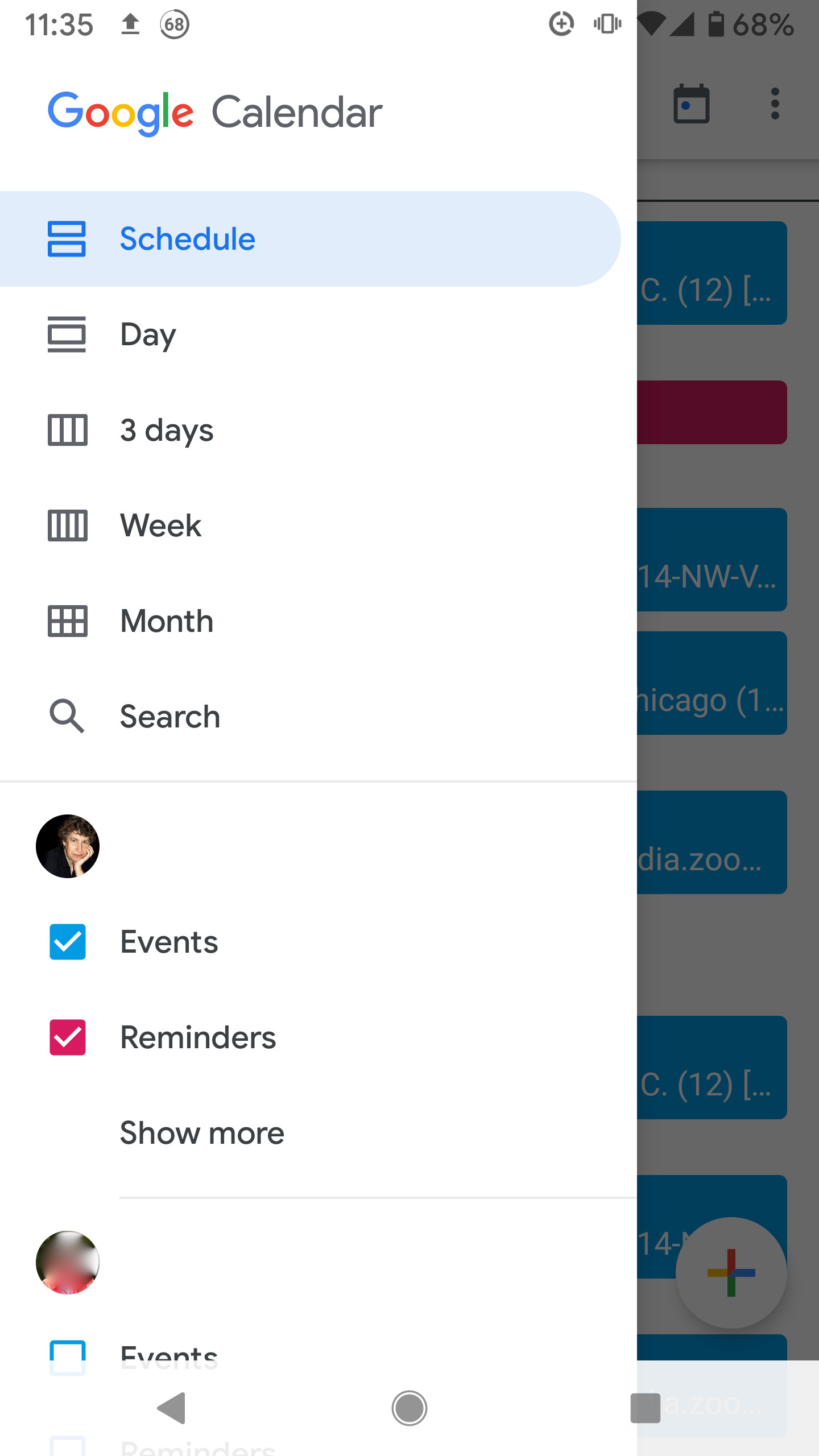This image is a screenshot taken from a mobile phone displaying the Google Calendar app. The current time, 11:35, is displayed in black text on a white background in the upper left-hand corner of the screen. On the upper right side, various mobile icons are present, including a battery icon at 68% charge. The main portion of the screen is occupied by the Google Calendar interface.

The app window covers about three-quarters of the screen, with the "Schedule" view selected, highlighted in blue. This selection sits on a white background. To the left, a vertical menu lists "Day," "3 Days," "Week," "Month," and "Search," each accompanied by small black icons. A small icon resembling a person’s head appears but is too small to discern details.

In the primary display area, there's a mix of event listings and settings. The "Events" option is clicked in blue, while the "Reminders" option is ticked in red. The "Show more" link is displayed underneath these selections. Another indistinct circle, possibly red and white, appears below the "Show more" link. The edge of another box labeled "Events" is visible but not selected.

At the bottom of the screenshot are several navigation icons: a gray back arrow, a circle in the center (likely the home button), and a square on the far right (possibly the recent apps button). There's also a faint watermark or semi-translucent text just beneath the events section, hinting at more Google Calendar settings or information.

The screenshot captures typical elements of the Google Calendar app interface, including navigation and scheduling options, all viewed through the lens of a mobile device.